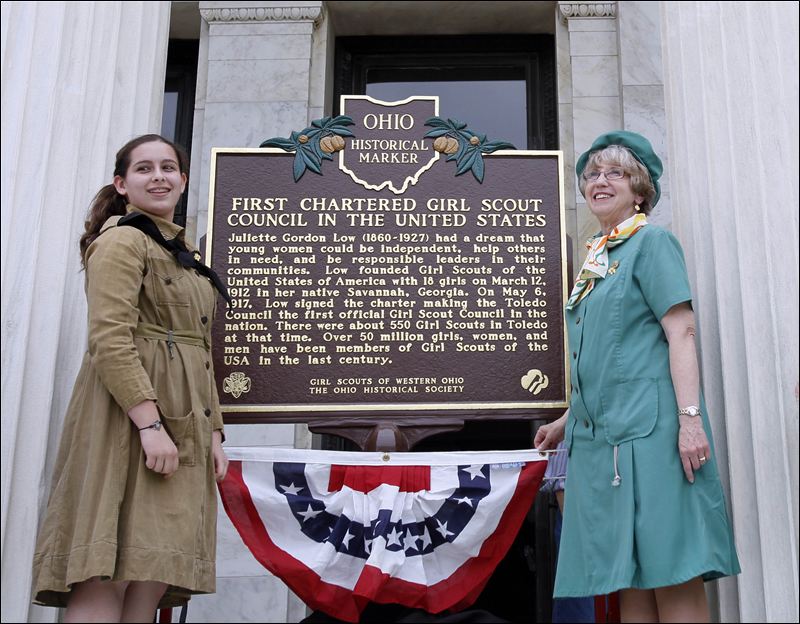This square photograph, taken in Ohio, captures a historical moment commemorated by an Ohio Historical Marker. In the image, two women stand on either side of the large bronze plaque entitled "First Chartered Girl Scout Council in the United States." The plaque, adorned with the shape of Ohio and intricate leaf designs, narrates the history of Juliette Gordon Low, who founded the Girl Scouts of the USA in Savannah, Georgia, on March 12, 1912, and signed the charter for the Toledo Council on May 6, 1917. This council became the first official Girl Scout Council in the nation. The plaque also highlights that over 50 million individuals have been members of Girl Scouts of the USA in the last century.

The women are dressed in traditional Girl Scout uniforms, evoking a sense of historical authenticity. The woman on the left, with brown hair tied in a ponytail, wears a light brown dress reminiscent of a Brownie uniform. The woman on the right dons a green Girl Scout dress, complemented by a yellow scarf and green beret. Detailed elements like a red, white, and blue bunting beneath the plaque, and the large white pillars of the building behind them, further emphasize the historical significance of the scene. The backdrop includes light bluish curtains and possibly a grand door, adding to the solemn and ceremonial atmosphere of the photograph.